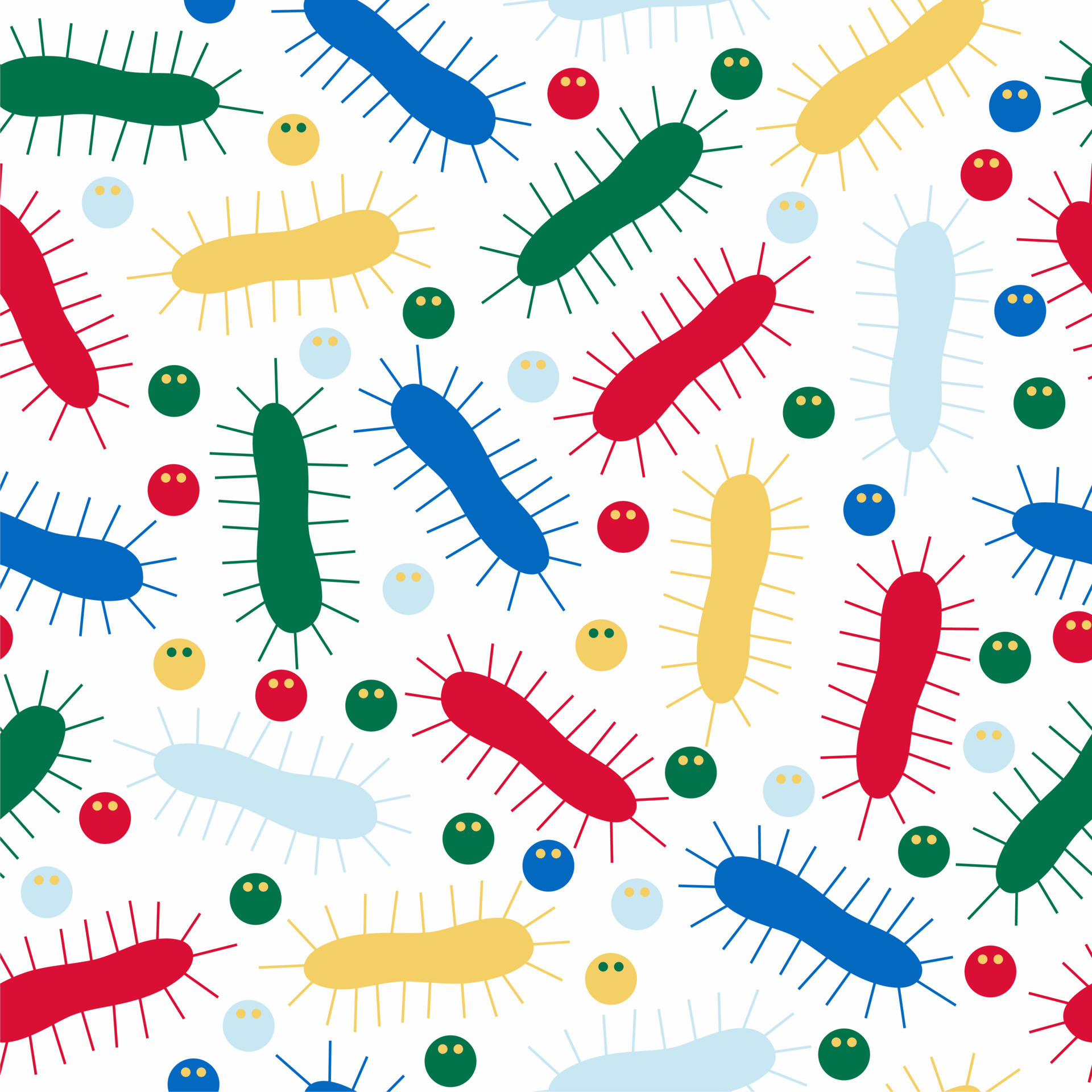The image showcases a vibrant, detailed drawing set against a completely white background, filling a square frame. It features numerous, colorful, tube-like shapes reminiscent of caterpillars or microscopic organisms. These shapes vary in color, including red, yellow, blue, light blue, green, and gold, and are adorned with spines or spikes. Interspersed among these larger shapes are smaller, circular objects, each with two yellow eye-like dots, resembling stylized depictions of germs or viruses. Arranged in a seemingly random, scattered fashion, the composition of the drawing is simplistic yet visually engaging, with some elements appearing partially cut off at the edges, suggesting a repeating pattern.